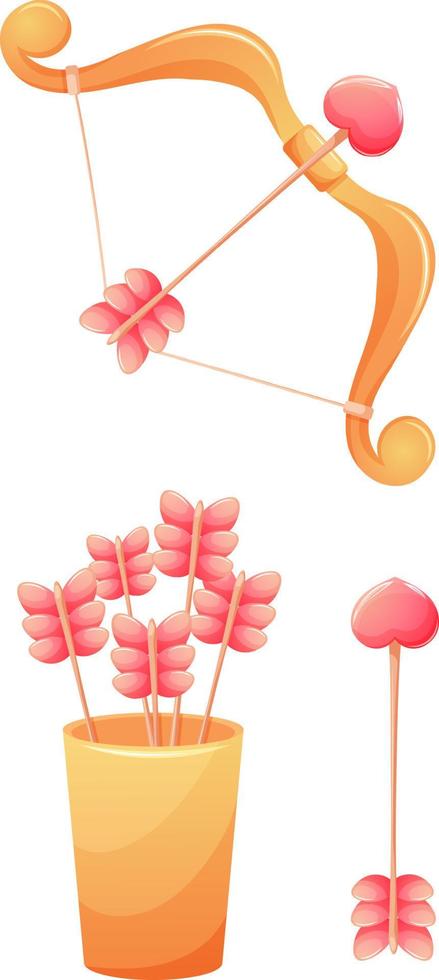The image is a colorful digital illustration with a Valentine's Day theme, showcasing Cupid's bow and arrow. At the very top, there is a shiny, green, and exaggerated compound bow pointed towards the upper right. A yellow string, pulled back to form a soft V shape, is connected to the bow. The arrow nocked on the string has a distinctive pink, heart-shaped tip instead of a traditional arrowhead. The arrow's shaft is wooden, and the feathers at the back are voluminous and fluffy, resembling butterfly wings stacked on each other. In the lower section of the image, there is a yellow, gold, orange, and red vase containing five additional arrows, all with pink heart tips and butterfly-like pink feathers. The entire scene is set against a wide background, emphasizing the romantic and whimsical nature of the illustration.